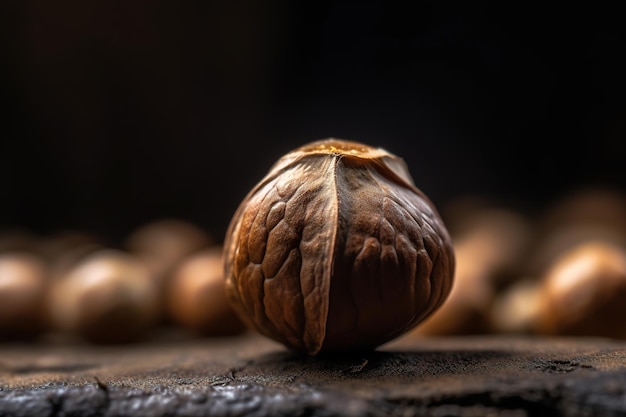This photograph showcases what appears to be a chestnut or a similar type of nut, positioned centrally as the main subject. The nut is round, with ridges running down its side, and bears a texture reminiscent of a walnut, though its shape and size deviate from the typical walnut's more oblong form. It rests on a surface that resembles either a slab of rock, an aged tree stump, or possibly a wooden piece. The background is solid black, enhancing the focus on the nut. Other nuts can be seen in the blurry, out-of-focus background, adding depth to the composition. The lighting comes from the left side, casting shadows on the right, indicating artificial indoor lighting rather than sunlight. The overall image has a slightly shiny and possibly AI-generated appearance, contributing to an almost surreal quality.